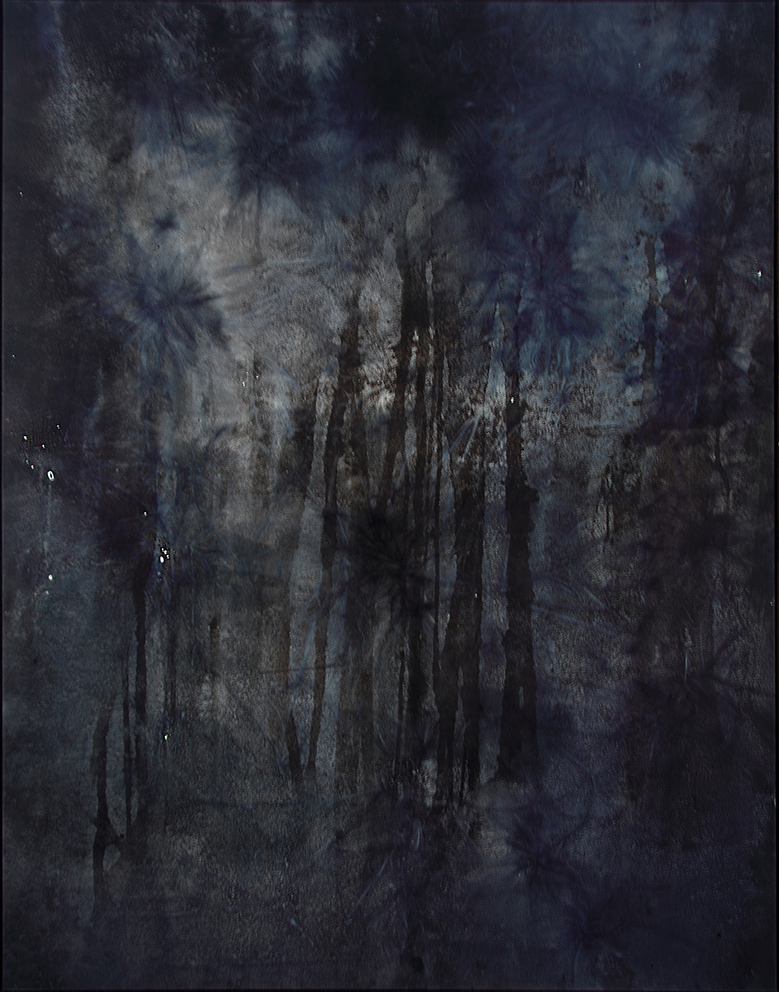The image appears to be an evocative oil painting portraying a hauntingly dark and mysterious nighttime forest. The overall palette is dominated by deep blues and blacks, interspersed sparingly with shades of gray and accented by subtle splatters of white, suggestive of distant stars. The painting features a series of tall, black vertical lines stretching about 80% of the way up and down the canvas, resembling tree trunks that cast shadowed reflections below them, creating an effect reminiscent of trees mirrored on water. The trunks are framed by splotches of dark blue on a lighter gray background, especially prominent towards the bottom, enhancing the depth and texture of the scene. Near the edges, the painting fades into pure black, enveloping the scene in an almost dreamlike, possibly nightmarish atmosphere. The composition is taller than it is wide, concentrating the viewer's attention on the central vertical elements that give the impression of a reflective, eerie forest at night.